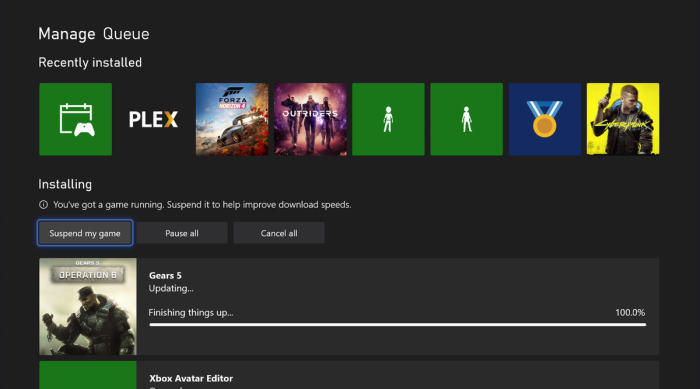The image depicts a dark black rectangular landscape interface, likely from a digital dashboard. In the upper-left area, slightly offset from the corner, there's white text that reads "Manage Q," with "Recently Installed" in a slightly smaller font below it. 

Under "Recently Installed," a series of eight small squares stretch from left to right, each displaying distinct images:

1. The first square features a green background with a white icon resembling a controller and a monitor.
2. The second square has a black background with the "Plex" logo in white, with the "X" partially in orange, representing the online media platform.
3. The third image appears to depict a tank or some sort of vehicle against a ground background, labeled "Forza" in black, suggesting a video game.
4. The fourth square shows three people in futuristic attire walking forward, labeled "Outriders," possibly indicating a movie or game.
5. The fifth and sixth squares are green with white icons of human figures in different stances; the left figure has its left leg straight with the right leg protruding, and the right figure displays the opposite stance.
6. The seventh square features a blue background with an illustrated gold medal, akin to an Olympic medal.
7. The final, eighth square has a yellow background with the word "Cyberpunk" in large yellow text. It shows an image of a man from the waist up, clad in a jacket, holding a pistol upwards with his head turned to the left.

Below the "Recently Installed" section, towards the left, white text indicates the status: "Installing." It advises, "You’ve got a game running. Suspend it to help improve download speeds." Three long rectangular buttons are shown, with the active one outlined in blue reading "Suspend My Game." The other buttons read "Pause All" and "Cancel All."

Further down is a larger rectangle highlighting the currently running game. It features a square image with a armored figure looking down, labeled "Operation 8" or "Operation B," followed by "Gears 5, Updating." Adjacent to this are progress indicators, including a bar labeled "Finishing Things Up" and a white line showing 100% completion.